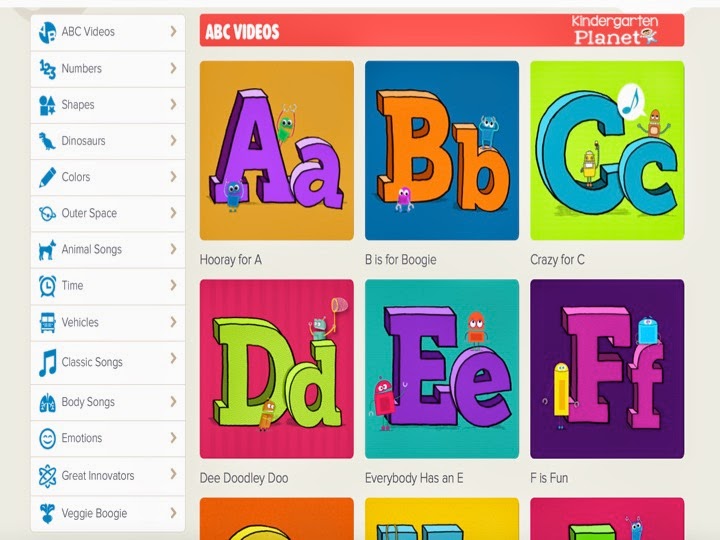The image showcases a vibrant and engaging learning website for children called "Kindergarten Planet." Dominating the top center of the page is a red banner; on the left side, it features the text "ABC Videos," while the right side proudly displays the website's name, "Kindergarten Planet," accompanied by a whimsical alien-like creature, presumably the site’s mascot.

On the left of the page, a vertical toolbar lists various sections of the website. These sections include: ABC Videos, Numbers, Shapes, Dinosaurs, Colors, Outer Space, Animal Songs, Time, Vehicles, Classic Songs, Body Songs, Emotions, Great Innovations, and Veggie Boogie. Each section name is clickable, directing users to the corresponding part of the website.

The main content area of the website showcases numerous colorful blocks, each highlighting a letter of the alphabet in both uppercase and lowercase forms. The first block has an orange background with purple letters displaying "A." Each letter block features the same format: an uppercase and lowercase letter, with an alien mascot either perched on or standing beside the letters. The blocks display a variety of background and letter colors, such as purple, orange, and light green, creating a visually stimulating and diverse learning environment.